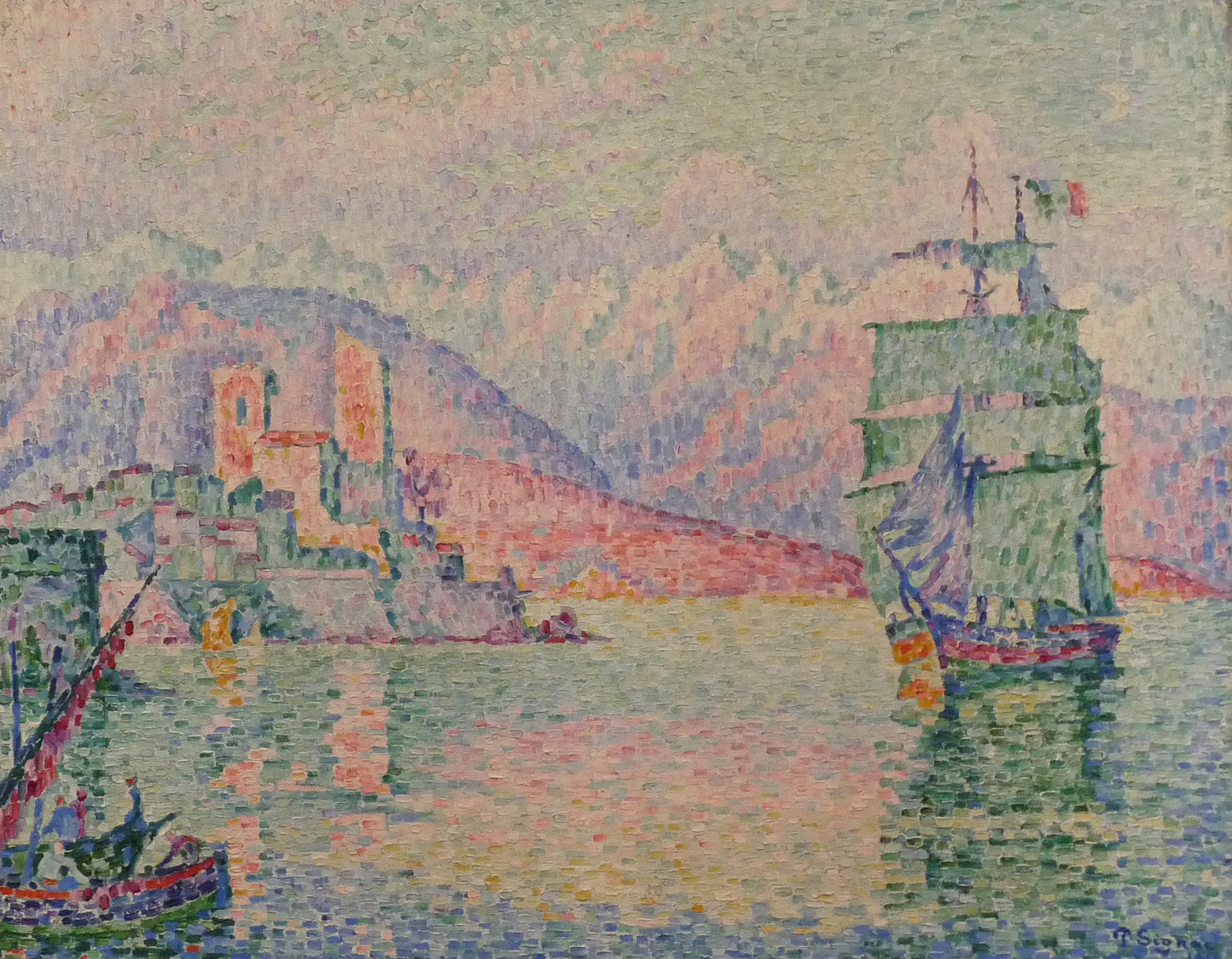This detailed, pointillist-impressionist painting, marked by its pastel hues of pink, purple, green, and blue, features a serene, flat body of water. Dominating the right side is a grand sailboat with green, tiered sails topped with green speckles and crowned with a sharp, purple point. The boat, painted in blue with a red streak down its middle, casts a shadow across the speckled water, which shifts in colors between green, blue, pink, and yellow. 

On the far left, a shoreline hosts a couple of light yellow buildings with red exteriors, one slightly taller than the other, featuring architectural elements like an arched top and a blue window. In front of these are more structures, predominantly green with hints of purple and yellow, and the front edge of another boat with people gazing towards the distant sailboat. The background showcases jagged, snow-capped mountains beneath a light green, clouded sky, adding to the painting's dreamy atmosphere. The artist's blue-inked signature, partly decipherable, is located in the bottom right corner. The entire scene is rendered in tiny strokes and points, blending together to create a hazy, dreamlike impression.